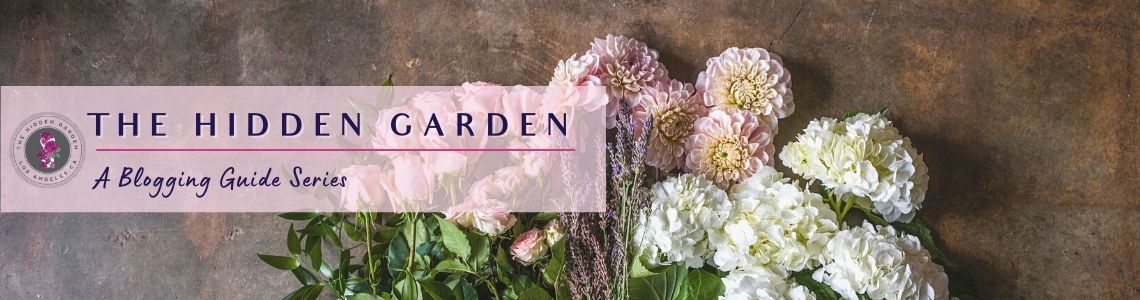The image is a banner ad featuring "The Hidden Garden," a blogging guide series. Set against a dark granite wall, the text overlays a background of both a rough brown wooden surface and an arrangement of flowers. The flowers, which include light pink and cream carnations, azaleas, and potentially roses, are scattered and surrounded by their green leaves and stems. To the left of the main text, there's a circular logo, blending somewhat with the floral background. The banner's text appears in pastel pink, harmonizing with the soft, pastel hues of the floral arrangement.